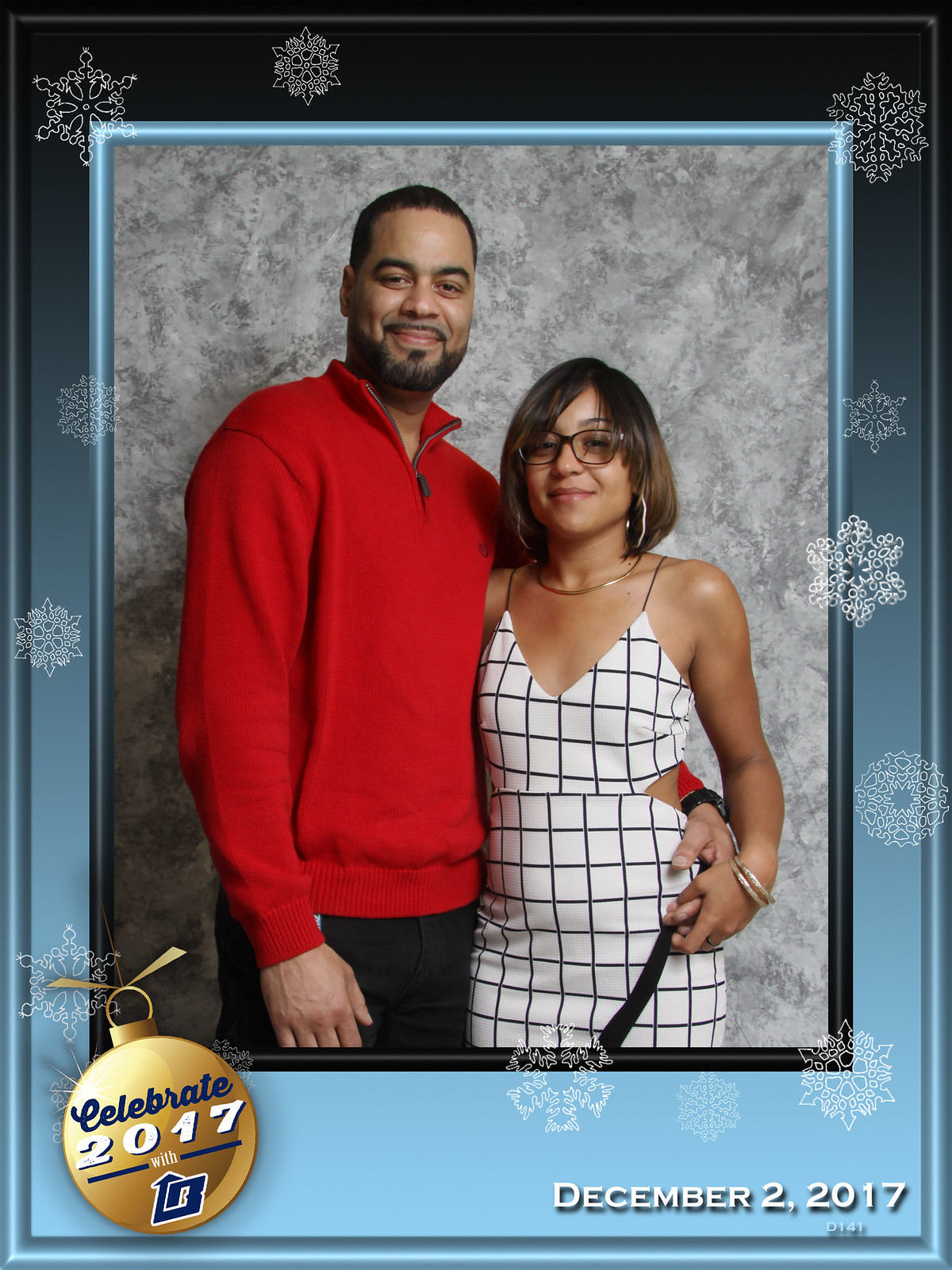The image is a detailed Christmas card from December 2nd, 2017, featuring a holiday scene with a young black couple posing against a gray, textured backdrop that has a sponge-painted effect. The card is bordered in a gradient from light blue at the bottom to dark blue-black at the top, adorned with white snowflakes and a gold Christmas ornament in the lower left corner with the inscription "Celebrate 2017 with." Below this, there's a logo that appears to resemble a 'B' with possible elements suggesting an 'L' in a modern graphic design with an arrow or small hat pointed upwards.

The man, standing on the left, is approximately 6 feet tall, wearing a red zip-up pullover and dark pants, with short black hair, a thin mustache, and a thin beard. The woman, standing on the right and held at the waist by the man, is about 5'4" or 5'5" tall. She dons a white dress with black line squares and spaghetti straps, complemented by a gold necklace, a gold bracelet, loop earrings, and eyeglasses. Her long dark brown hair drapes elegantly to her shoulders. Both individuals are captured arm in arm, exuding a charming and festive aura.  Below the image, in the lower right-hand corner, "December 2nd, 2017" is inscribed.